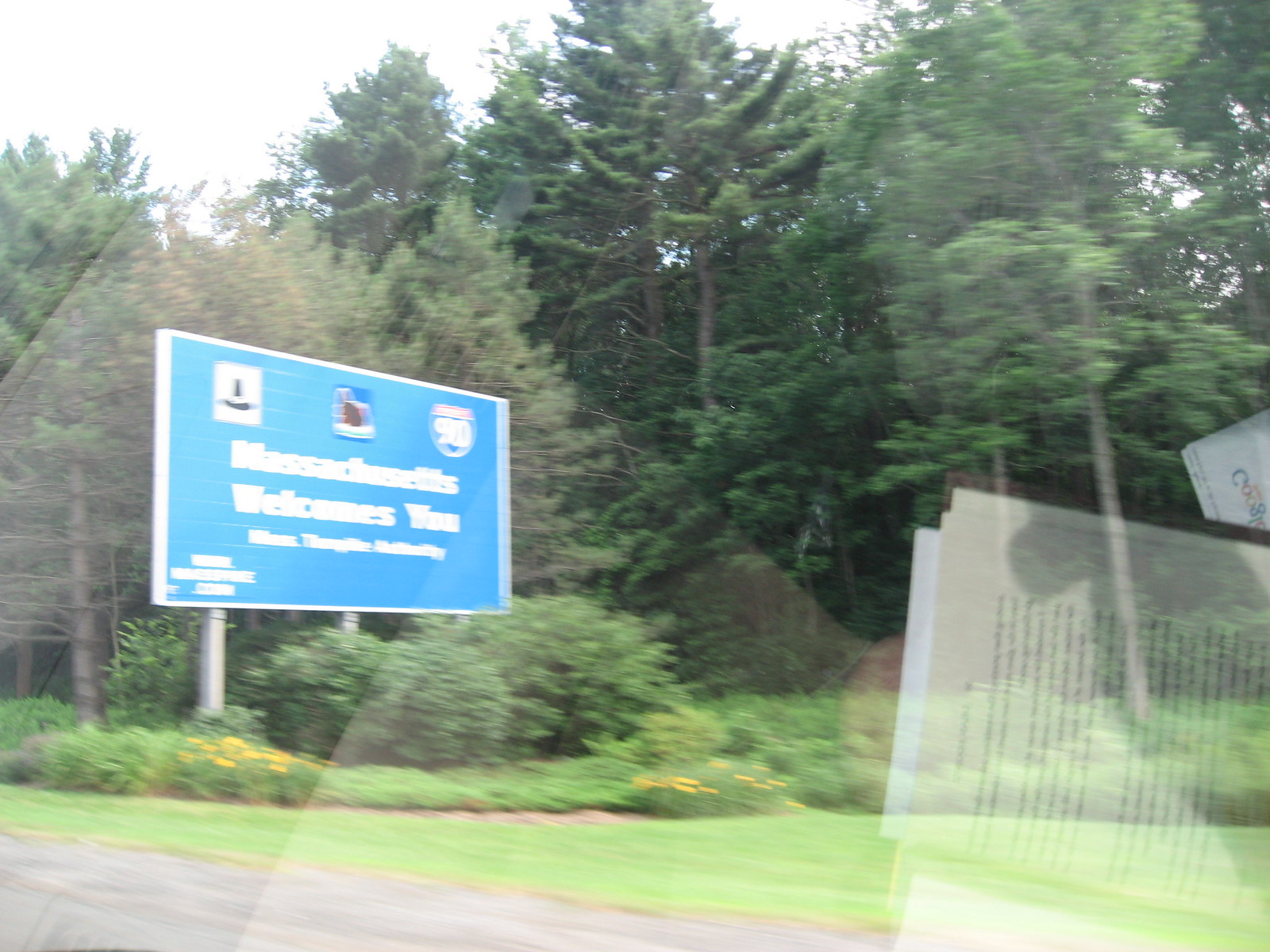This image captures a blurry scene through the window of a moving vehicle. Central to the photograph is a prominent blue rectangular sign reading "Massachusetts Welcomes You" in large, clear text. Despite the blur, the sign features additional elements including a website URL in the bottom left corner, although the exact text is indistinguishable. The top right of the sign displays a badge with the number "90" and the image of an animal, accompanied by a distinctive shape that resembles a witch's hat. The sign is situated in a forested area, surrounded by tall trees and bushes, with a green grass field in the immediate vicinity. Reflected in the vehicle's window, one can discern an open book and a visible webpage on a device, indicating the presence of a passenger engaged with reading and browsing the internet.